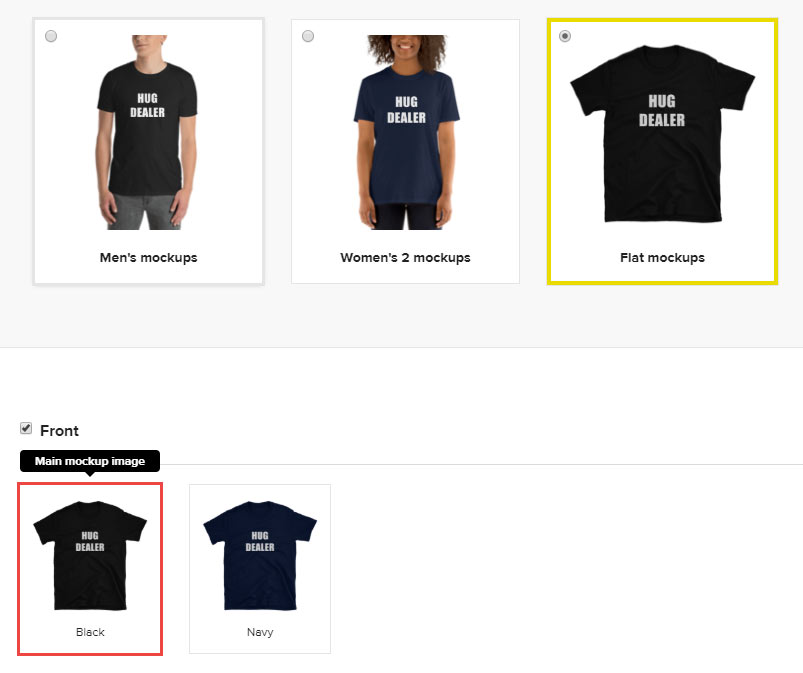The image showcases a webpage dedicated to selling t-shirts emblazoned with the playful slogan “Hug Dealer,” a humorous twist on the phrase “Drug Dealer.” The webpage is designed to display various mock-ups of the t-shirts, which come in black and navy with bold, white text. The word "Hug" is emblazoned in large capital letters ("H-U-G"), placed above the word "Dealer," also in all caps ("D-E-A-L-E-R"), ensuring the text stands out prominently against the darker shirt colors.

On the left side of the image, there is a clickable section labeled "Men's Mock-Ups." Within this section, a partial view of a male model is shown, cropped from the nose down to the thighs, wearing one of the “Hug Dealer” t-shirts. Adjacent to this, another section labeled "Women's Mock-Ups" features an African-American woman smiling brightly, dressed in black pants and a navy “Hug Dealer” t-shirt.

Further to the right, there is an image of an unworn t-shirt highlighted with a yellow rectangle, designated as "Flat Mock-Ups." This image emphasizes the shirt as a standalone product.

Towards the lower part of the page, additional options are provided. There is a section that reads "Front," "Main Mock-Up Image," and indicates the color options available, with a red rectangle highlighting the black t-shirt, though navy is also an option.

This clearly designed webpage effectively highlights the whimsical “Hug Dealer” t-shirts, offering potential buyers multiple viewing options through mock-ups and emphasizing the product's color choices and standout design.